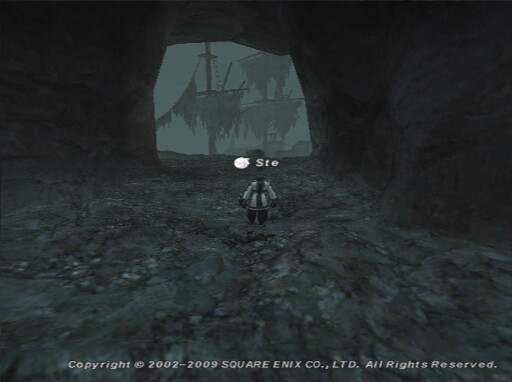In this slightly horizontal image, likely a capture from a video game, a solitary figure stands at the very center, appearing minuscule against their surroundings. The character is clad in a long, white coat featuring a distinct dark stripe down the middle, paired with black pants. They face an expansive opening in a solid rock wall, which frames the scene beautifully. Through this vast opening, the distant silhouette of a ship with tattered sails can be discerned, adding a touch of mystery and adventure. At the bottom of the image, italicized white text reads: "Copyright 2002-2009 Square Enix Co., Ltd. All Rights Reserved," providing a formal acknowledgment of the creator and timeframe of the content.